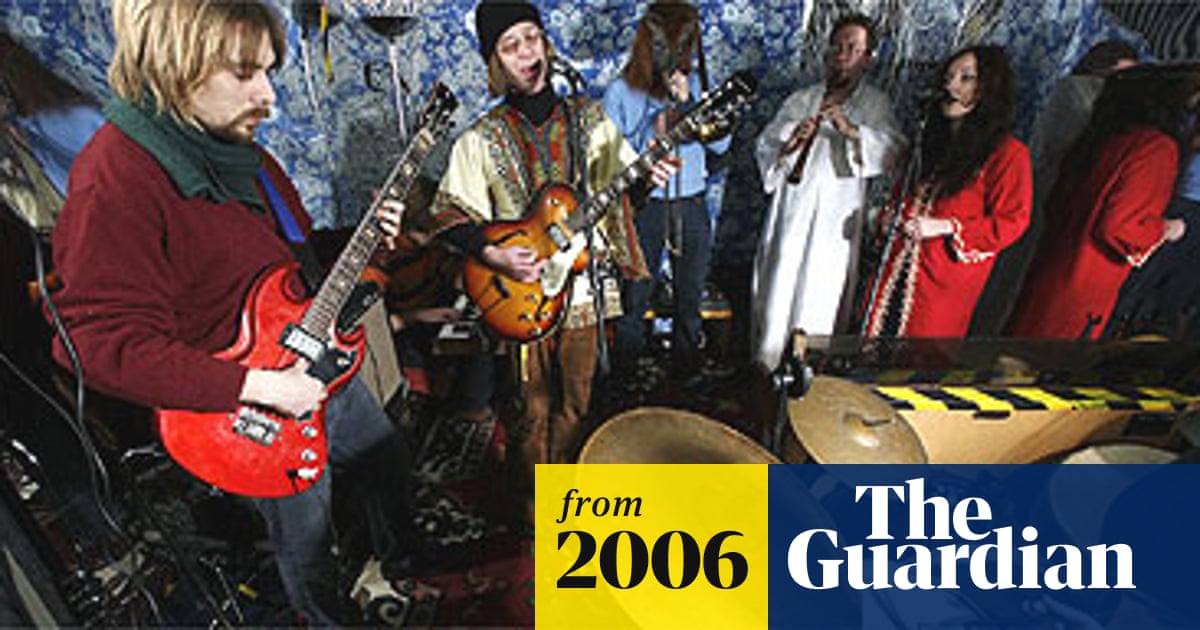The image, possibly from a 2006 article or advert in The Guardian, presents a detailed front-view shot of a band performing on stage with a blue and white floral backdrop. From left to right, the composition displays:

- A man on the far left in a red jacket playing a red guitar.
- Next to him, another man is both singing into a microphone and holding a guitar.
- To his left, a person with long hair in a blue shirt also sings into a microphone.
- Adjacent to them is a man dressed in a solid white robe, playing a woodwind instrument resembling a clarinet.
- On the far right, a woman wearing a vibrant red dress, who has long black hair, is singing.

A mirror behind the performers reflects the woman in the red dress. In the foreground, partially visible, is a drum set with cymbals, suggesting a complete band setup. The words "From 2006, The Guardian" are noted in the bottom corner of the image, indicating its source. The ensemble's attire and the detailed stage setting imply a possible performance at a fundraiser or an autumn/winter music festival, likely leaning towards a folk music genre.